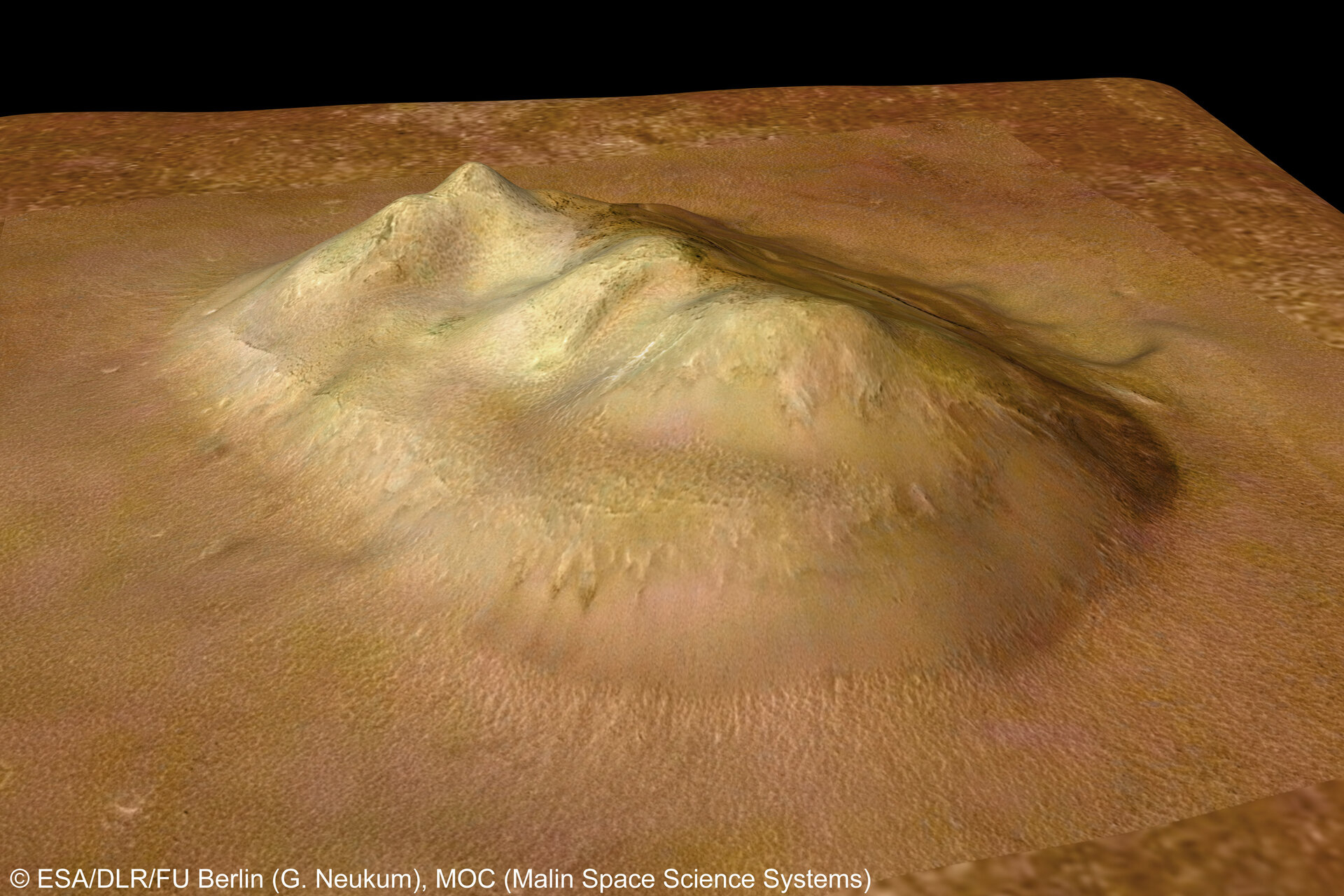This is a three-dimensional recreation of a tall mountain with three distinct peaks rising dramatically from a Martian desert landscape. The mountain's slopes exhibit mottled shades of green and very pale orange, contrasting with the expansive, sandy plains that eventually give way to a darker, rocky terrain in the distance — though this detail might be an artifact of the composite photography. The photograph, with somewhat unclear and overlaid sections forming a mosaic, is copyrighted by ESA/DLR/FU Berlin (G. Neukum) and Malin Space Science Systems, indicating its origin and credit. The predominant hues of gold, brown, and pitch black further emphasize the harsh, rugged beauty of the Martian surface.